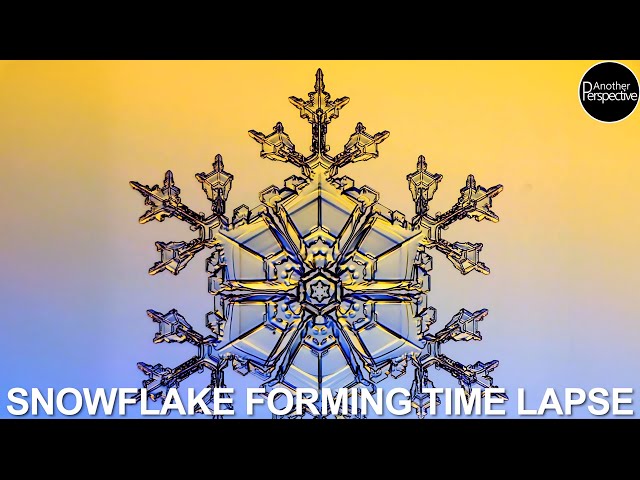This image appears to be a frame from a widescreen video presentation, potentially a thumbnail for an online video. The frame is bordered by narrow black strips along the top and bottom, enhancing its cinematic feel. Dominating the frame is a detailed pixel art depiction of a large, transparent snowflake crystal, vividly set against a gradient background that transitions from yellow at the top to blue at the bottom. The snowflake is intricately designed, capturing the complexity of an ice crystal in a microscopic view. Along the bottom of the frame, white uppercase text with a shadow effect reads "SNOWFLAKE FORMING TIME LAPSE." In the upper right corner, a black circle with a white border contains the phrase "ANOTHER PERSPECTIVE" in white text, likely representing the producer or company behind the video.